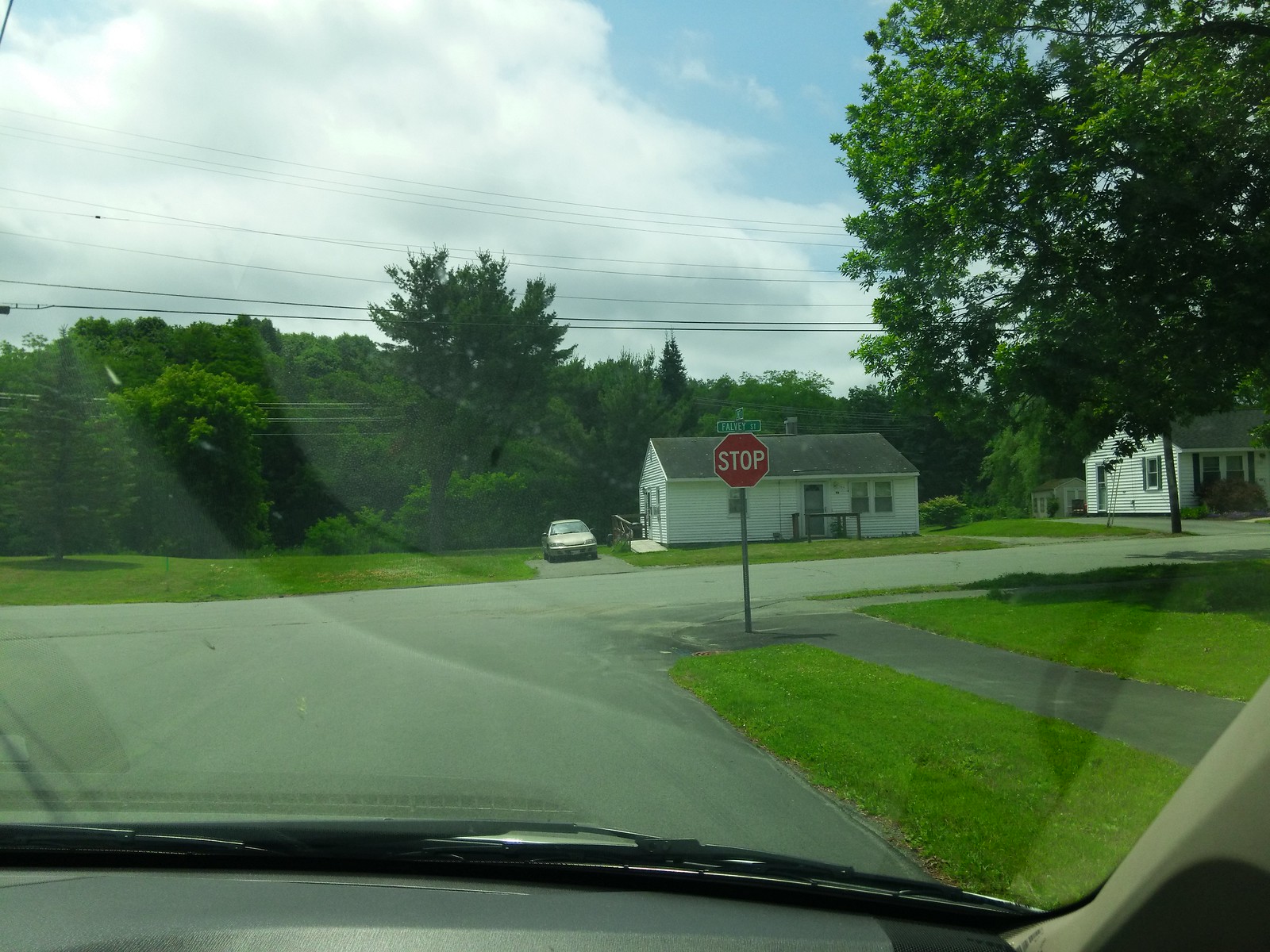The photograph captures an outdoor scene from inside a car, looking through the windshield. The car is approaching a stop sign at the end of a road, which is framed by a green street sign above it. The windshield shows shadows and reflections, including that of a black windshield wiper, indicating the perspective from within the vehicle. 

In the upper portion of the image, a very blue sky is dotted with a large, fluffy white cloud toward the left. The backdrop features a lush green area filled with trees of varying shades. To the right of the scene stands a prominent tree with abundant green leaves. Below the trees, the landscape transitions to a well-maintained lawn.

In the background, two white houses are visible, suggesting a quaint neighborhood setting. The house on the left appears modest and possibly dates back to the forties or fifties; it has a gray roof and a gold car parked in its adjacent stone driveway. The house on the right is slightly more ornate but shares a similar style. Both houses are accompanied by power lines running above them, adding to the suburban atmosphere.

Foreground elements include a strip of cut green grass and a dark gray or black asphalt sidewalk that runs parallel to the road. The overall composition is dominated by the road itself, an asphalt path that varies from light to dark gray, leading directly toward the stop sign.